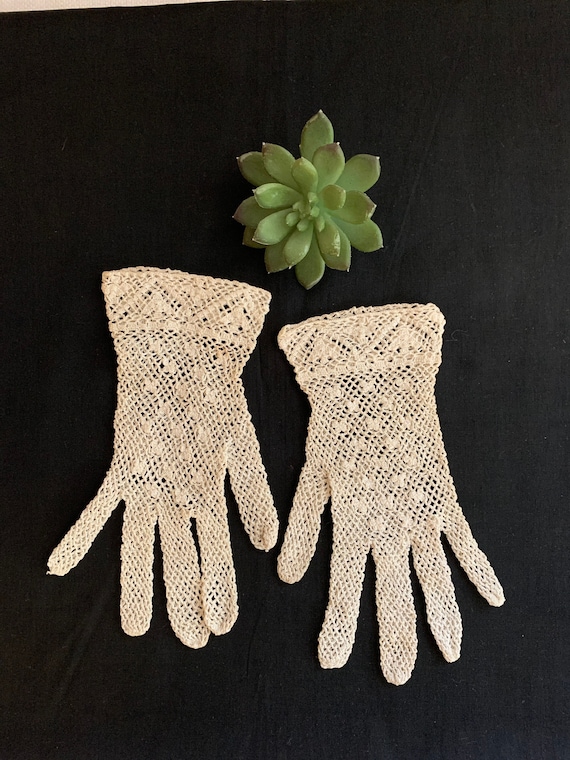The photograph features two ivory, lace-like crochet gloves and a smaller green succulent plant, all set against a predominantly black background that appears to be some sort of velvet material. The background shows a slight fringe of cream or white at the top left corner, where the black material doesn't cover the entire frame. The intricate gloves, delicate yet made from thicker crochet string, display vintage craftsmanship with patterned cuffs and possibly butterfly motifs. Positioned with the fingers and thumbs facing downward, the left glove sits slightly higher than the right. Although well-preserved and antique in appearance, the gloves exhibit minor snags on the pinky and have somewhat misshapen, elongated fingers. The succulent, resembling a flower with numerous small leaves, is located just above the gloves at the center of the composition.